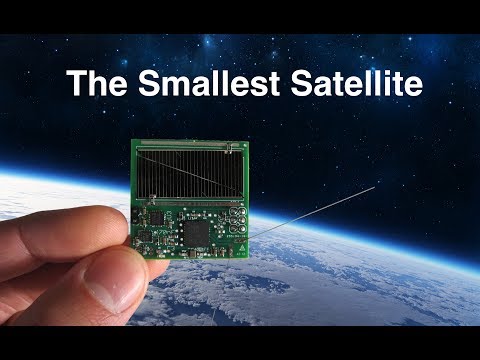The image is an intricate photo illustration featuring a close-up of a person's left hand, identifiable by the visible thumbnail and first two fingers, delicately holding a small, square-shaped green microchip. The microchip is detailed, showcasing a large black and grey chip on its top surface, surrounded by several smaller black and silver components, including circuits and resistors. An antenna or large grey line extends to the right of the chip, adding to the complexity of the device. Positioned prominently in the background is a majestic space scene featuring a starry sky and a close-up view of a planet or moon, which is distinguishable by its fuzzy blue atmospheric border. This celestial body, possibly Earth, floats against the dark expanse dotted with stars. Just above the microchip, white text reads "The Smallest Satellite," suggesting the image may serve as an advertisement or promotional label. Above the planet, a solitary object appears to be flying in a straight trajectory, blending seamlessly into the cosmic backdrop.